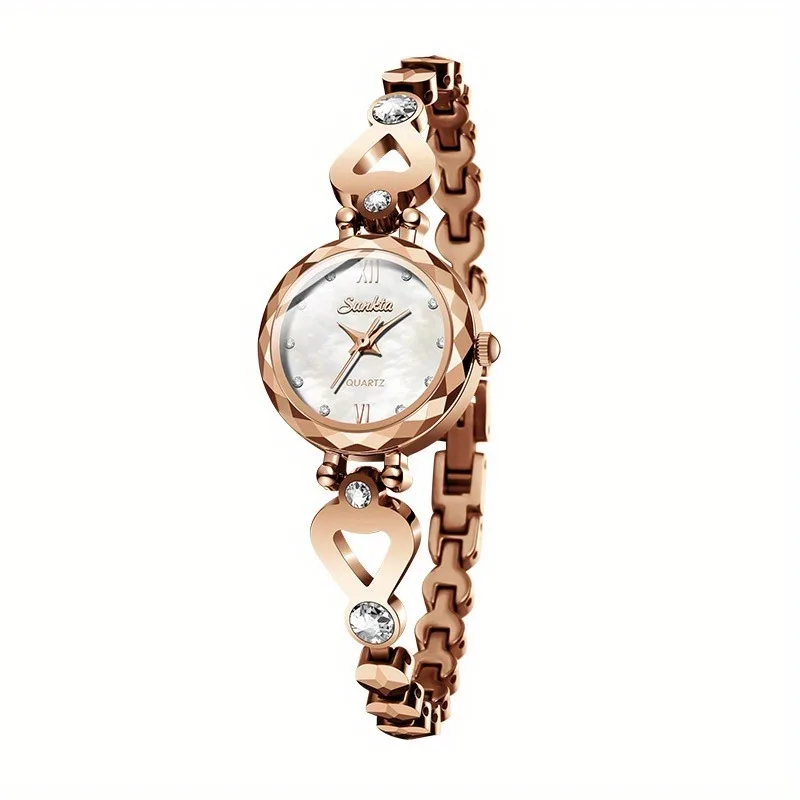The image appears to be a computer-generated advertisement for a luxurious female wristwatch, characterized by its elegant rose gold color and intricate design. The band of the watch consists of thin interlocking links, resembling small wrenches with curved patterns, giving it a refined, chain-like appearance. Nestled within the band are small circular diamond accents that add a touch of sparkle.

The face of the watch is predominantly white, enclosed by a clear glass cover. Prominently displayed at the top and bottom of the watch face are the Roman numerals XII and VI respectively, while the other hours are marked by tiny diamond circles. The hour, minute, and second hands are painted in a combination of silver and rose gold, enhancing the overall theme of opulence.

A distinct feature of the watch is the heart-shaped clasp adorned with diamonds at both the top and bottom, linking the watch face to the band. The brand name, likely "Sun Surkta" or "Sankhya," is inscribed on the front of the watch face, along with the term "quartz," emphasizing its precise timekeeping mechanism.

The entire scene is set against a plain white background, ensuring that every detail of the watch is highlighted, from the elegant, three-dimensional band to the sophisticated watch face.